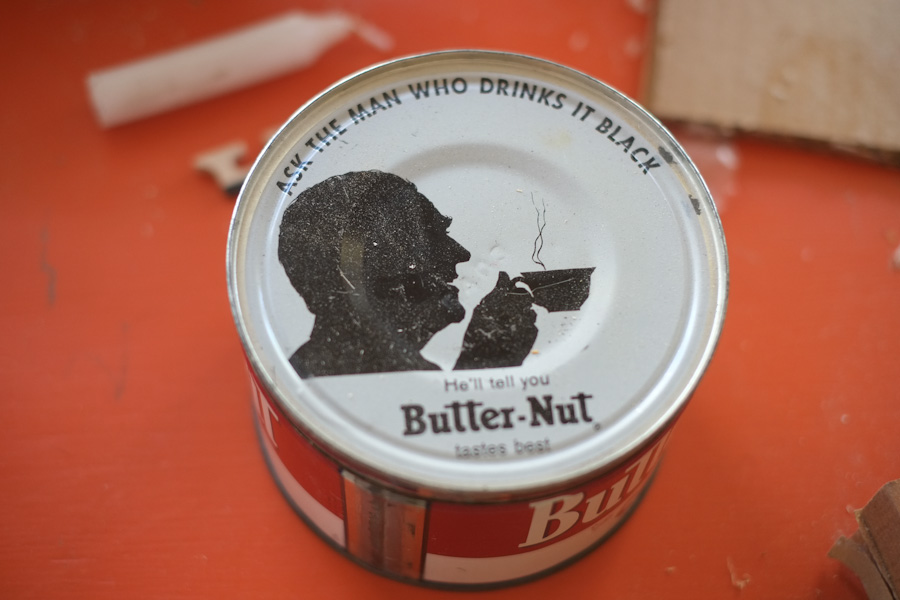This vibrant color photograph captures a small, circular, silver-topped tin can resting on a bright orange surface. The can, primarily white with red accents, prominently features an illustration of a man's silhouette sipping a steaming cup of coffee, accompanied by black, curving text above that reads, "Ask the man who drinks it black." Directly below the man's image, more text states, "he'll tell you Butternut tastes better." On the side, the can displays a bold red banner with the white letters "BU" followed by a white banner. Surrounding the can, the orange surface is scattered with bits of fluff and thread. In the background, a white candle lies in the top left corner, while a tan piece of cardboard occupies the top right.